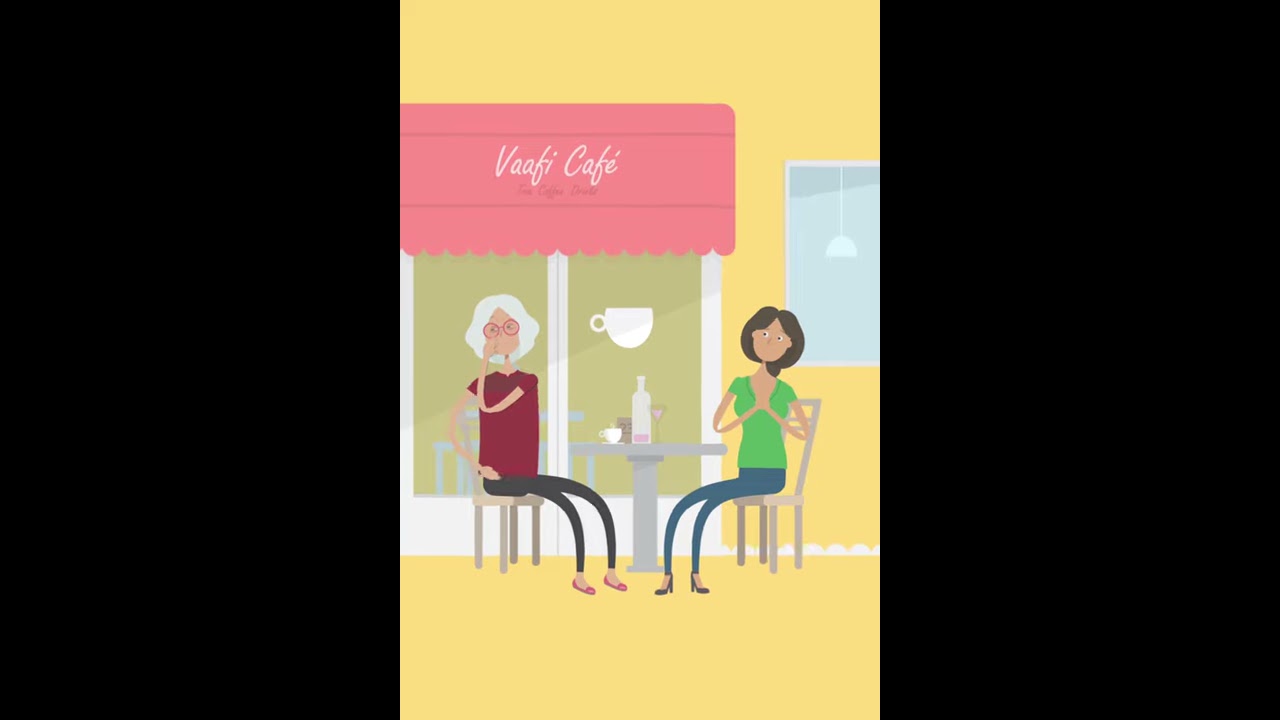In this vibrant, cartoon-style digital artwork, we see an inviting scene set outside the Vafi Café. The café itself has a bright yellow wall and prominently features a red canopy above a white-framed window with glass. In front of this window, a grey circular table serves as the focal point where two women are seated, one on the left and one on the right. 

The woman on the left sports white hair and red glasses, complementing her red short-sleeved T-shirt and black pants. Opposite her, the woman on the right has long black hair and brown skin, wearing a green short-sleeved T-shirt with blue pants. Both women appear to be enjoying their drinks—likely coffee—with a bottle of wine also set on the table, suggesting a leisurely, relaxed atmosphere. 

The café's name, "Vafi Café," is visible in the background, adding to the scene's charm. The floor of the seating area shares the café's yellow hue, while black empty space frames the left and right sides of the image, focusing attention on the central characters and their surroundings. A stylized coffee cup design is also present on the window, reinforcing the café theme. This image captures a lively and cozy outdoor moment in a digitally-animated, hand-drawn style.